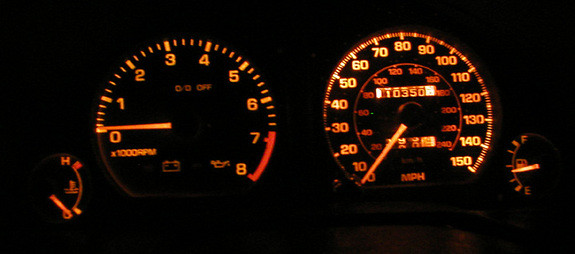The image showcases the instrument panel of a vehicle, prominently presenting gauges and displays in a classic layout reminiscent of 1980s and 1990s models. 

At the far left, the fuel gauge indicates a level slightly below half. On the far right, the temperature gauge reads at the baseline level, denoting a cold engine since the vehicle is turned off. Centrally positioned, the tachometer and speedometer dominate the display. The tachometer, which measures the engine's RPM, ranges from 0 to 8,000, with sections marked in white and the red zone starting at 7,000 RPM. The speedometer, featuring increments of 10 miles per hour, spans from 0 to 150 mph and includes finer dash marks between major intervals for precise readings. 

The total mileage of the car, displayed in the middle of the speedometer, is currently noted at 10,350 miles. All gauges and displays feature illumination, primarily in white, enhancing visibility, with red lighting used for certain high-alert zones, such as the upper range of the tachometer.

Overall, the dashboard is minimalist yet functional, embodying the straightforward design aesthetics of late 20th-century automobiles.